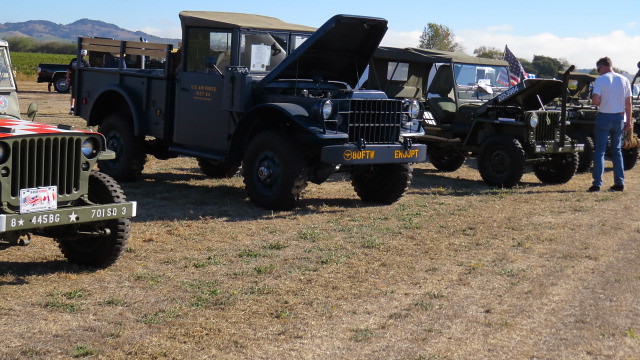The image depicts a lineup of military-style vehicles parked on a sparse dirt road with patches of green grass. In the foreground, several Jeeps and pickup trucks, including a distinctive blue pickup truck with wood paneling and yellow lettering, are parked stationary. One Jeep, which is checkered red and black, has its hood open. A green Jeep also has its hood open. Next to this green Jeep, a man dressed in a white t-shirt and blue jeans is inspecting the engine. The vehicles feature various colors including camouflage, blue, olive green, and some have military identifiers like "8445 BG 701 SD3" and "60 FTW EXEMPT," with one vehicle even displaying an American flag. In the background, you can see trees and brush, leading up to a stunning purple and gray mountain range under a beautiful blue sky. There are also some low clouds hovering above the mountains, enhancing the scenic backdrop. Additionally, a black truck is partially visible behind the lineup of military vehicles.